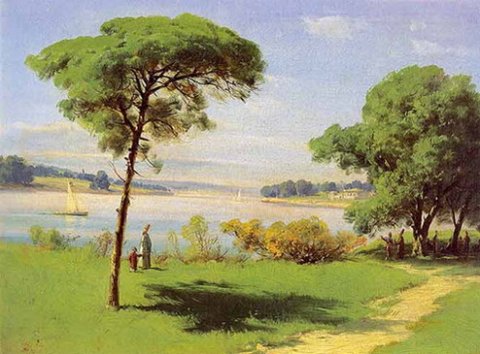This painting depicts a serene park scene on a sunny day, centered around a small lake bordered by green grass and tan walking paths. In the foreground on the right, there's a large tree with brown trunks and dark green leaves under which some people are gathered, possibly wearing red and blue. To the left, a taller individual and a child stroll by the shore, near a standalone tree. Dominating the middle of the image is a light blue lake with a sailboat featuring white sails. The background showcases an expansive sky with soft white clouds. Distant trees and open fields mark the horizon, completing this gentle and soothing portrayal reminiscent of Van Gogh's style.